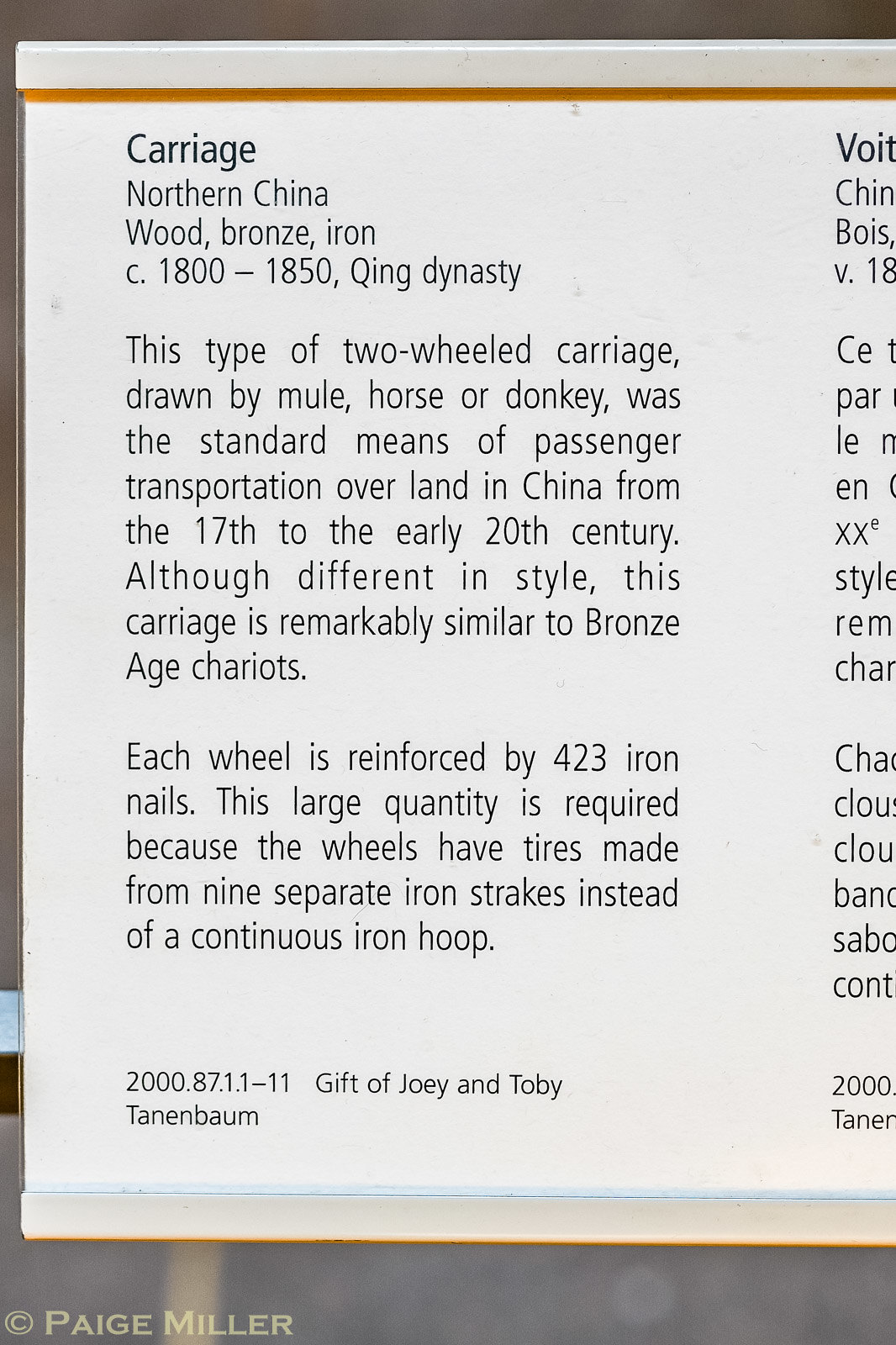The image features a close-up of a museum sign centered in the frame, detailing a historical carriage from northern China, dating back to the Qing Dynasty, circa 1800-1850. The sign provides extensive information about the two-wheeled carriage, which was typically drawn by a mule, horse, or donkey and served as the standard means of passenger transportation overland in China from the 17th to the early 20th centuries. Despite stylistic differences, the carriage bears a striking resemblance to Bronze Age chariots. Notably, each wheel of the carriage is fortified with 423 iron nails, a design necessity due to the tires being fashioned from nine separate iron strakes rather than a single continuous iron loop. The text on the sign appears in black and white, with visible colors in the image including white, black, orange, brown, tan, and gray. It also mentions the copyright belonging to Paige Miller. The overall setting indicates the sign is part of a museum exhibit, despite the carriage itself not being visible in the photo.